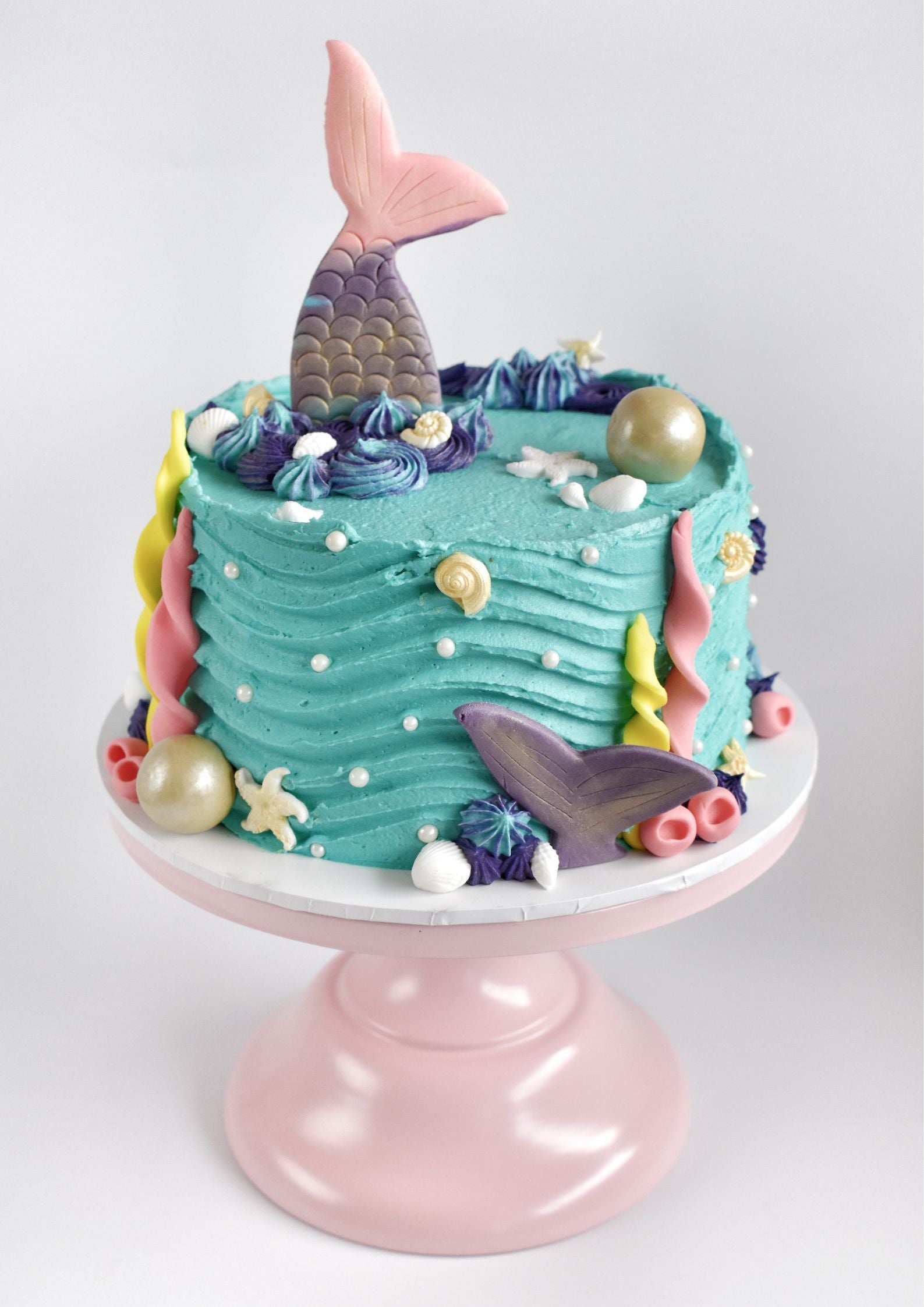This image features a uniquely detailed birthday cake with a mesmerizing fish-themed design, prominently displayed on a pastel pink pedestal, which elegantly contrasts with the plain white background. The cake itself is a vivid turquoise and brims with intricate oceanic decorations. Scattered across its surface are seashells, starfish, and spiral fondant shaped like seaweed, all adorned in a variety of colors, including pink, beige, yellow, purple, and blue. A distinctive feature is the pink fish half-emerging from the top, alongside another fishtail decor element. Pearlescent accents, resembling gumballs, embellish the cake, with one large pearl at the top adding a touch of glamour. The cake's sides mimic gentle waves, enhancing its underwater aesthetic. Based on its size, the cake seems perfect for an individual serving, seamlessly integrating numerous marine-inspired details into a small, captivating confectionary masterpiece.